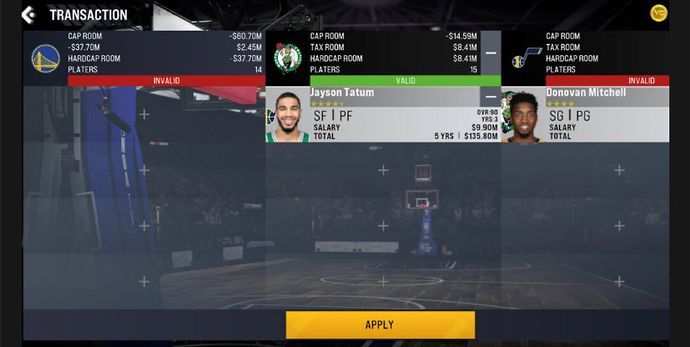The image depicts a screenshot of a website displayed on a desktop with a black background and white text. At the top of the screen, there is a white back arrow, followed by the word "Transaction." The website is divided into three distinct sections or tables.

The first table contains a profile section and states "Cap Room" with a figure showing a negative balance of $60.7 million. A red bar labeled "Invalid" indicates something is wrong with this transaction.

The second table presents similar categories, including "Cap Room" and additional text details about "Hard Cap Room." This section features a green bar labeled "Valid," suggesting this transaction is acceptable. Additionally, there is an image of a man named Jason Tatum along with a rating and salary information.

The last table also includes "Cap Room" and other related categories but shows a red bar labeled "Invalid." This section features an image of another individual, Donovan Mitchell.

In the background of these three tables, a stadium is visible, likely a basketball stadium. At the bottom of the screen, there is a feature labeled "Apply" written in black ink over a yellow band.